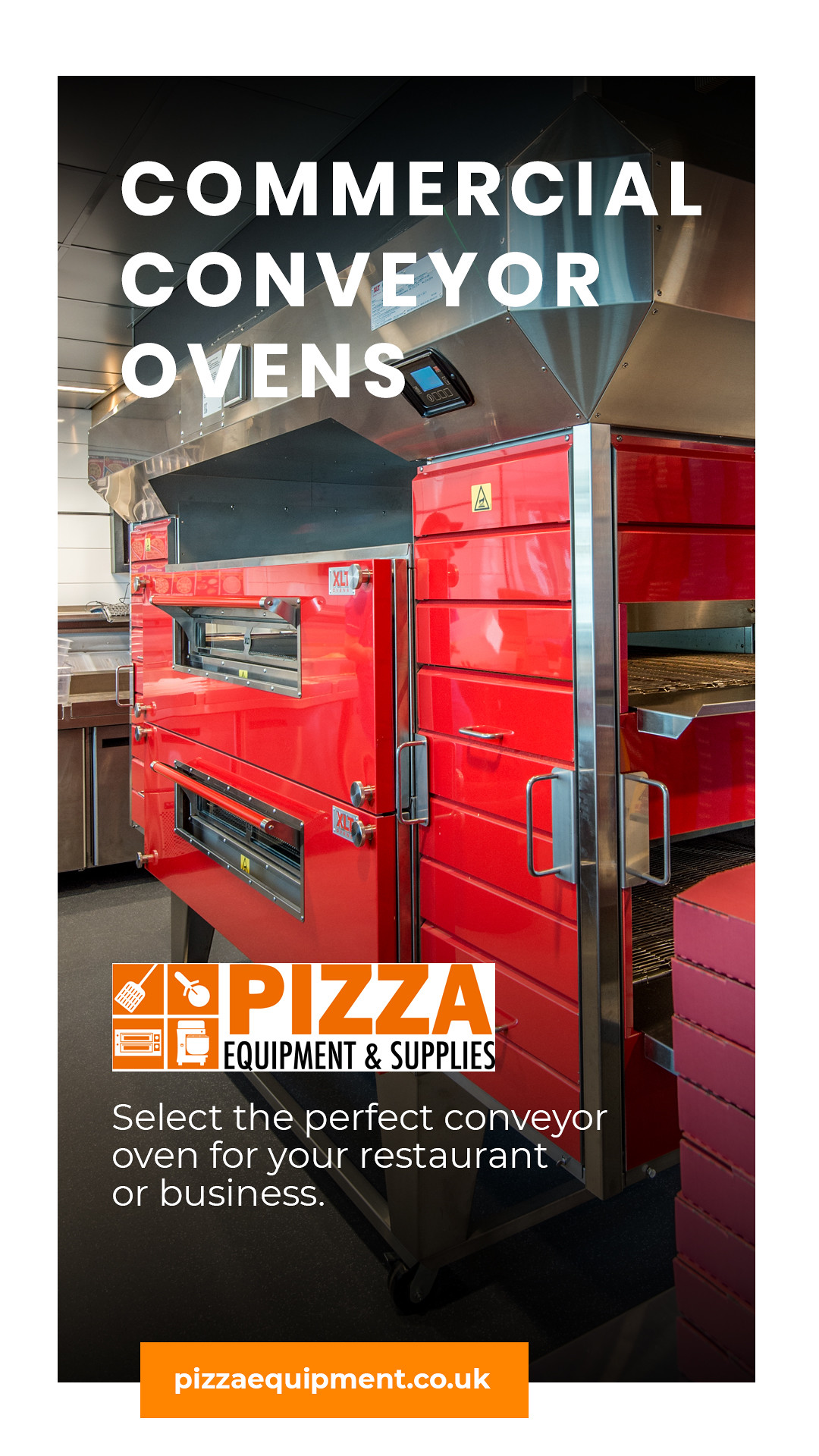This vertically oriented advertisement features a detailed color photograph of a large, red commercial conveyor pizza oven with shiny black and silver stainless steel handles and trim. The oven, which appears to have two individual baking chambers, operates on a conveyor belt system where pizzas are inserted on one side, cooked as they travel through, and emerge fully baked on the other side. Text at the top of the image reads "Commercial Conveyor Ovens" in white block letters, followed by "Pizza Equipment and Supplies" positioned centrally with accompanying small logo images. Further down, it instructs viewers to "Select the perfect conveyor oven for your restaurant or business." An orange block of text at the bottom of the image displays the website, "PizzaEquipment.co.uk."